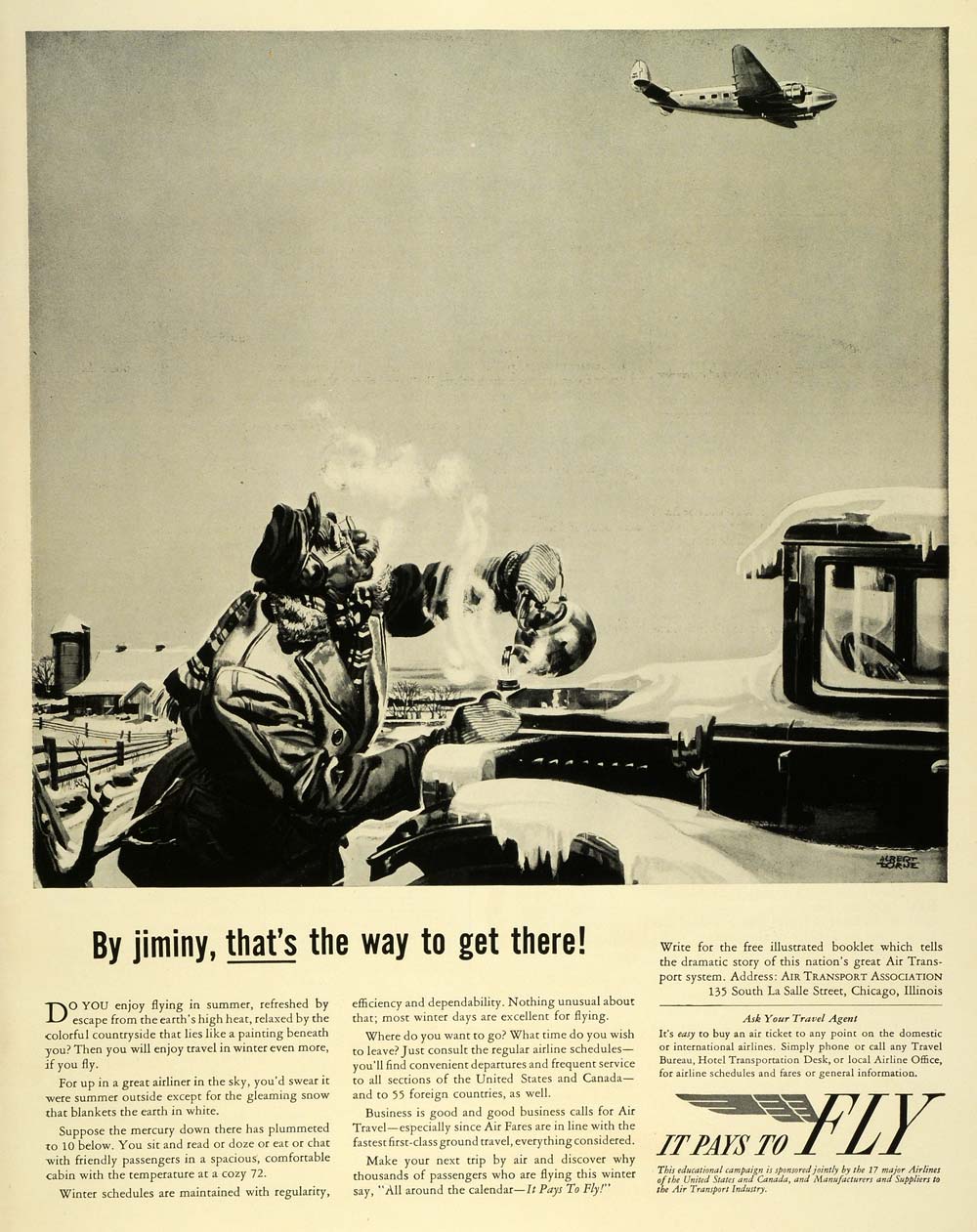The image is an old vintage advertisement with a black and yellow color scheme. The central illustration is in black and depicts a man in winter standing outside near a house and a barn. The man, snow-covered, is holding a tea kettle and appears to be pouring steaming liquid into a cup, possibly to defrost a car engine. To the right of the man is a black truck, likely a 1950s Chevy, also covered in snow. In the background, there's a long wooden fence typical of a ranch and a farm with a silo. Above the man, an airplane is flying towards the right side of the image. Below this scene, the text reads "By Jimminy, that's the way to get there," and in the lower right-hand corner, it states, "It Pays to Fly." The bottom part of the image contains three columns of black text.